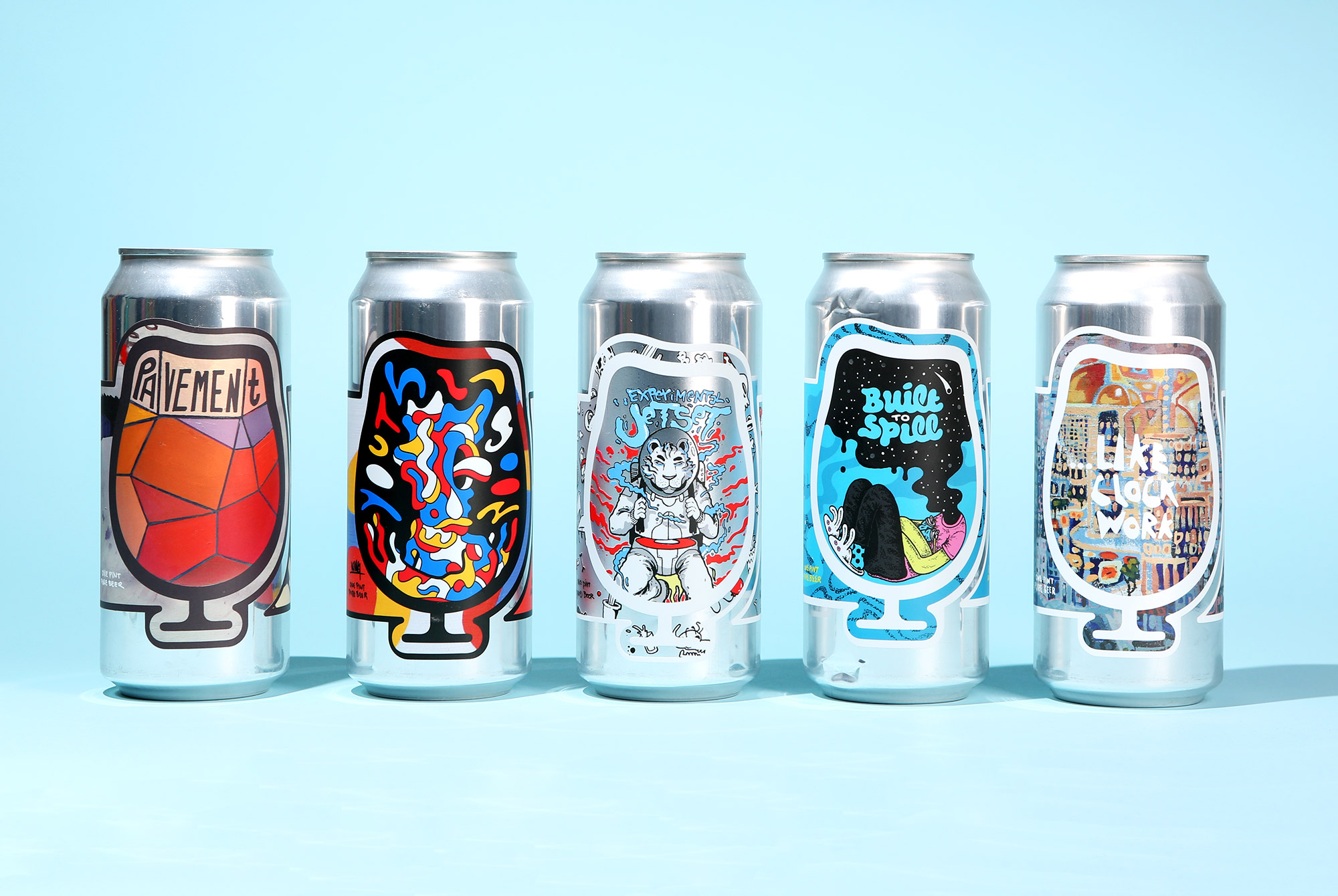The image features five unique, retro-styled beer cans. Each can, mostly white and cylindrical in shape, showcases distinct and colorful artwork. Starting from the left:

1. The first can displays a vibrant wine glass filled with red, orange, and slightly linked geometric shapes like triangles and squares. Above the wine glass, three small yellow squares spell out "Pavement."
2. The second can features another wine glass adorned with intermingling white, red, and blue lines, creating an abstract and dynamic pattern.
3. At the center is a striking can with a white tiger or snow leopard dressed in a spacesuit, poised as if ready to fight.
4. The fourth can prominently exhibits the phrase "Built to Spill" in chunky blue letters, accompanied by a visually striking image of a black sky cascading into the form of a person.
5. The last can in the sequence reads "Like Clockwork" in white letters and is surrounded by what appear to be book-like illustrations.

All the cans exude a fun, hip, and retro aesthetic, making them eye-catching and distinctive.